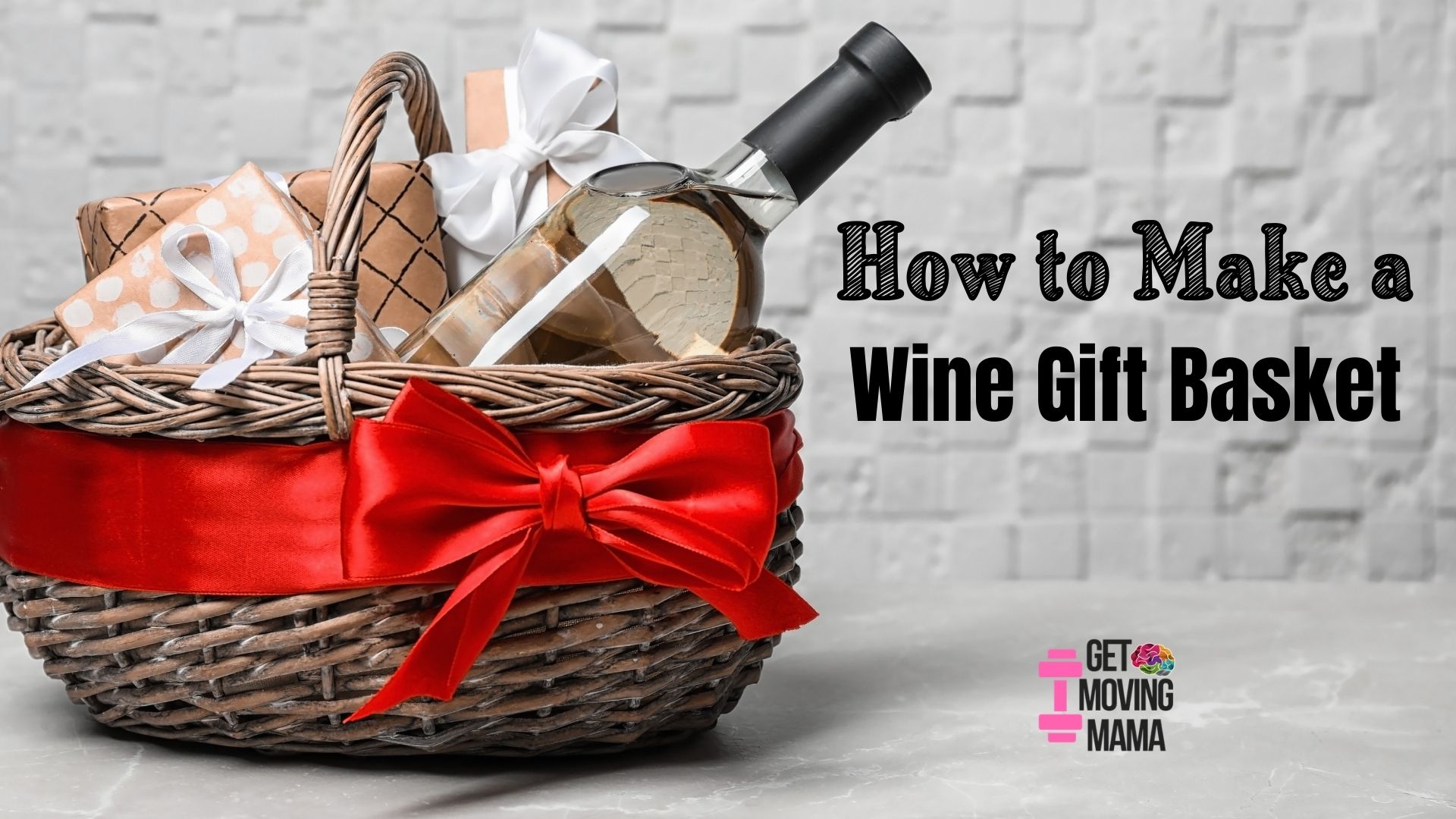The image showcases a wicker gift basket with a braided handle, adorned with a prominent red ribbon tied in a bow. Inside the basket, there's a clear bottle, possibly wine although the liquid is transparent, capped with black. The basket also contains three distinctively wrapped gifts: one beige with white polka dots and a white ribbon, another light brown with a checked pattern, and a taller beige package with a big white bow. The background features a white brick wall and a white table. The caption "How to Make a Wine Gift Basket" is written in black letters on the right. At the bottom, the label reads "Get Moving Mama," accompanied by a pink dumbbell on the left and a flower-like pinwheel on the right.